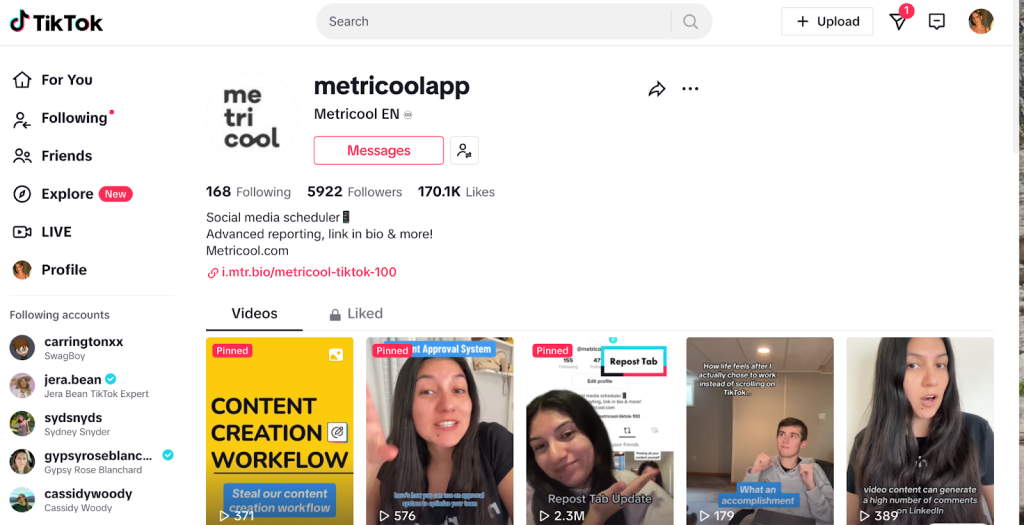The screenshot displays the main page of TikTok, specifically the Metricool profile, on a desktop interface. Metricool's profile highlights their role as a social media scheduler and analytics provider. The account has 168 followed accounts, 5,922 followers, and a total of 170,000 likes. Metricool appears to collaborate with content creators to optimize their social media presence. The profile features pinned videos, including a content creation workflow guide and an update about a new TikTok feature. On the left side of the screen, navigation options like For You, Following, Friends, and Explore are visible, typical of the TikTok desktop layout.